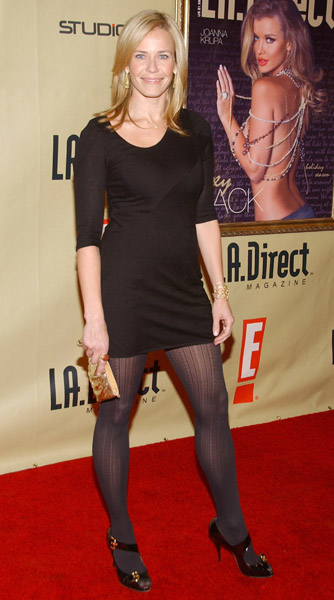A striking photograph captures a beautiful woman standing confidently on a red carpet, facing forward and smiling directly at the camera. She is dressed in a chic black mini dress paired with dark pantyhose and stylish black heels. Her radiant shoulder-length blonde hair frames her face, accentuated by long earrings. The woman carries a gold purse in her right hand and has delicate jewelry adorning her wrist. The backdrop behind her is a gold-colored wall featuring black text that reads "L.A. Direct Magazine" along with a red exclamation mark logo of the company "E". To the upper right of the image, there is a large poster of Juliana Krupa posing bare-backed with jewelry, adding a touch of glamour to the scene. The overall setting suggests an upscale event sponsored by L.A. Direct Magazine.